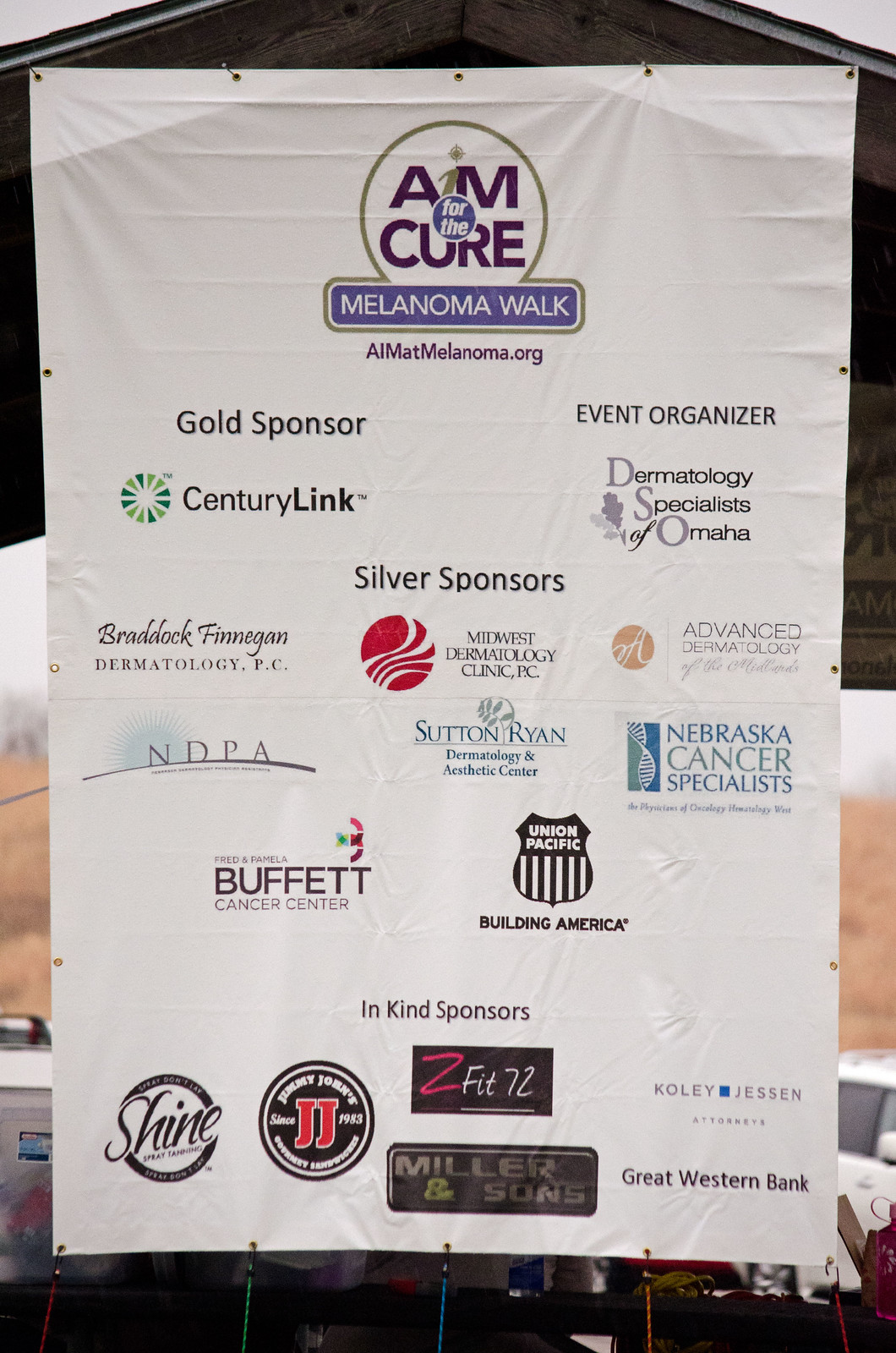The image showcases a white banner hung from an awning, prominently displaying the "Aim for the Cure Melanoma Walk" event. The central upper part of the banner features the event's logo: a green circle with the words "Aim" and "Cure" in the center, flanked by "For the" written in white on a blue button within the circle, and a blue rectangle underneath reading "Melanoma Walk." The banner, made of stretched white plastic, lists the event's sponsors in descending order of prominence. At the top, "Gold Sponsors" and "Event Organizers" are highlighted, including CenturyLink and Dermatology Specialists of Omaha. Following in the "Silver Sponsors" category are entities such as Braddock Finnegan Dermatology and Midwest Dermatology Clinic. The "In-Kind Sponsors" listed at the bottom feature brands like Jimmy John's, Z Fit, and Great Western Bank, accompanied by their respective logos. The overall backdrop is white, emphasizing the detailed listing of sponsors and their contributions to the event.